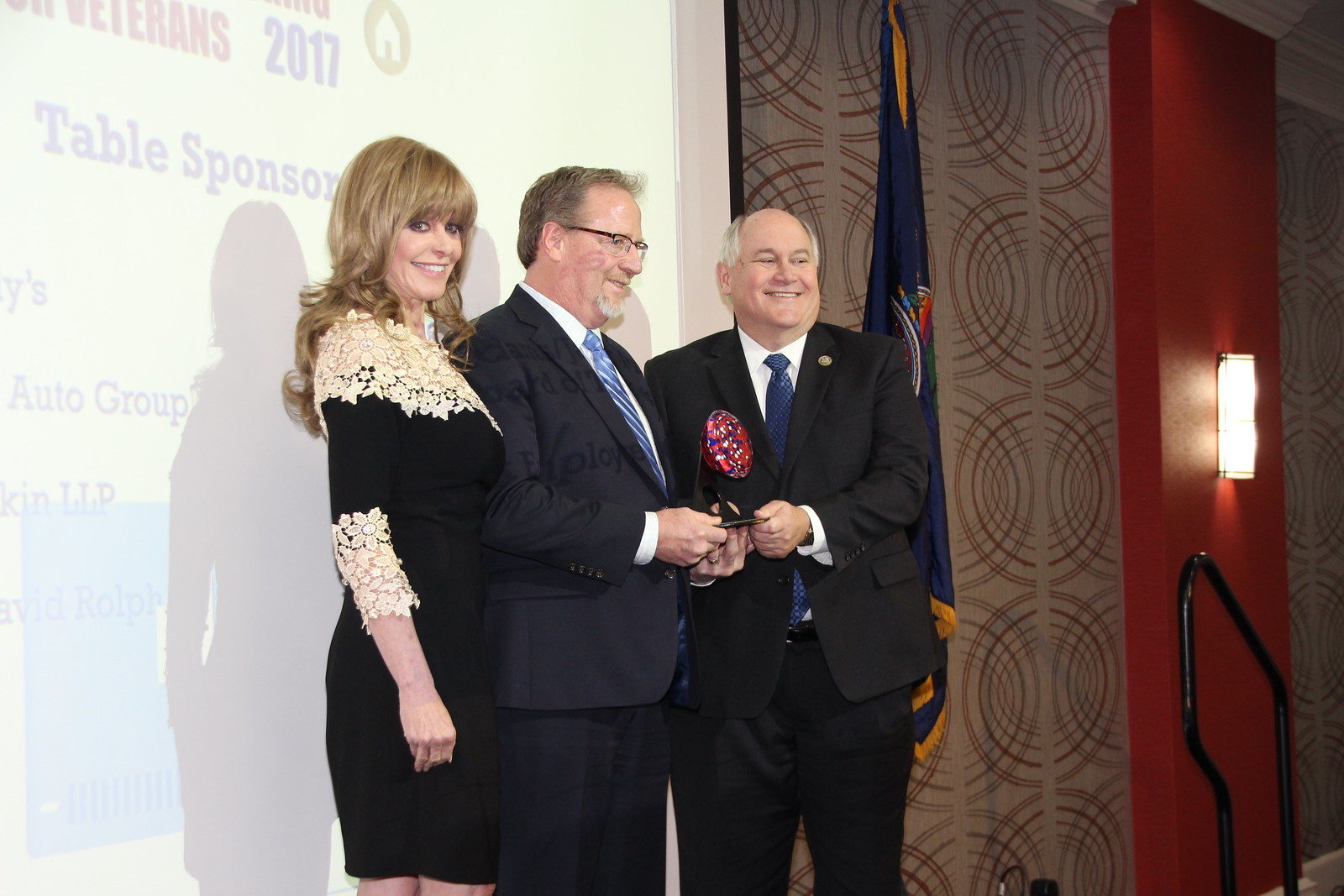In this photograph, we see a formal award presentation taking place indoors. At the center of the image, three middle-aged individuals are prominently featured. 

On the left, a smiling Caucasian woman with blonde hair stands out. She is wearing a dark, form-fitting dress adorned with lace detailing at the neckline and sleeves. To her right is a man with a short brown hair, gray beard, and glasses. He is dressed in a dark suit, white shirt, and blue tie. The man is holding an award with a black base and a red top. Facing them is another man, who is balding and heavyset, also clad in a dark suit with a blue tie and white shirt. 

Behind the trio, the background features white walls and a softly illuminated screen with partially visible text, including “Veterans 2017,” suggesting the nature of the event. Additionally, there are beige, brown, and orange curtains draping down, further emphasizing the formality of the setting. The banner displaying "table sponsor" hints at the organized setting, while the textured wallpaper on one side adds to the indoor ambiance. Despite the lack of readable text, the joyous expressions and attire of the individuals highlight the significance of the occasion.